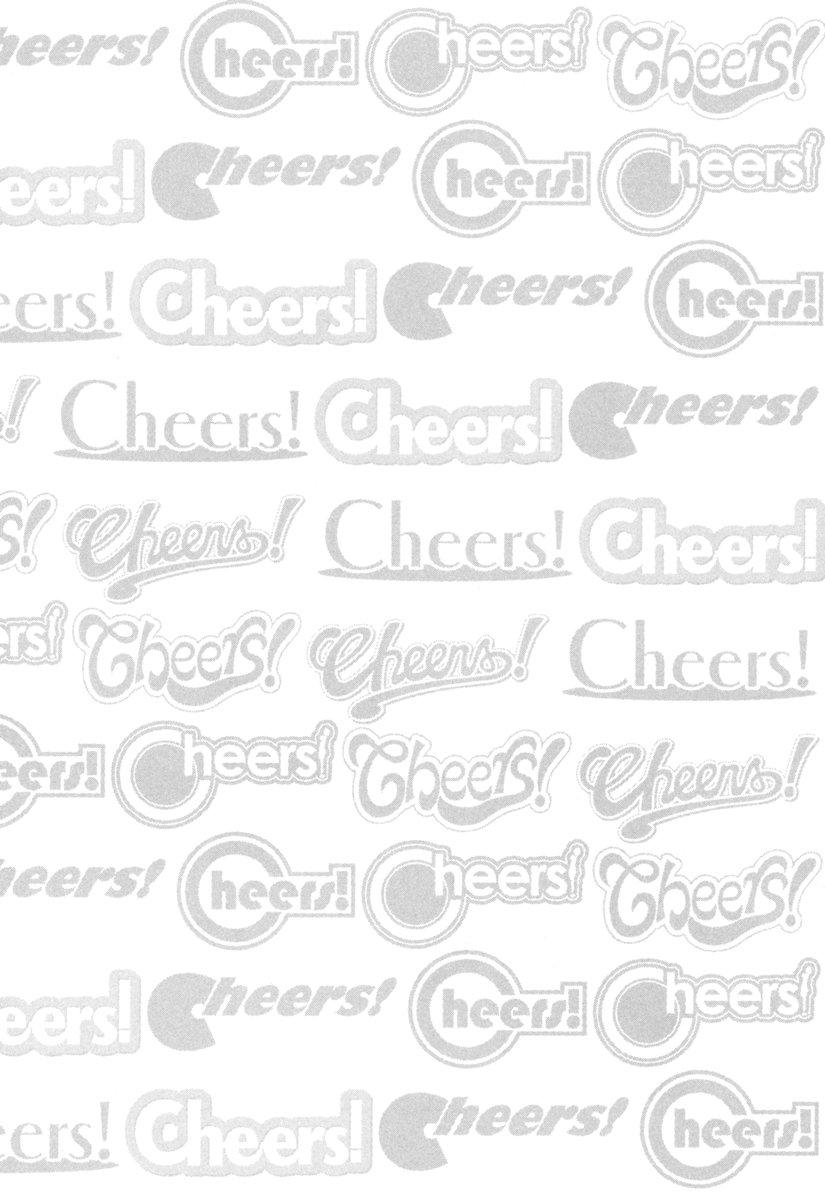The image features a white background filled with over 40 distinct logos, all of which spell the word "CHEERS!" in various styles and fonts. The text is uniformly gray, with each instance of "CHEERS!" presented in countless different typography styles—ranging from basic block text to semi-cursive scripts evocative of beer logos. Some iterations feature bold lettering, while others are adorned with decorative elements such as elongated tails beneath the letters or circular designs incorporating the "C" and "H." The logos are arranged in a repeating pattern, where each line showcases "CHEERS!" multiple times, often alternating styles to create a diverse visual tapestry. Each logo prominently includes an exclamation point, adding to the celebratory feel of the composition.